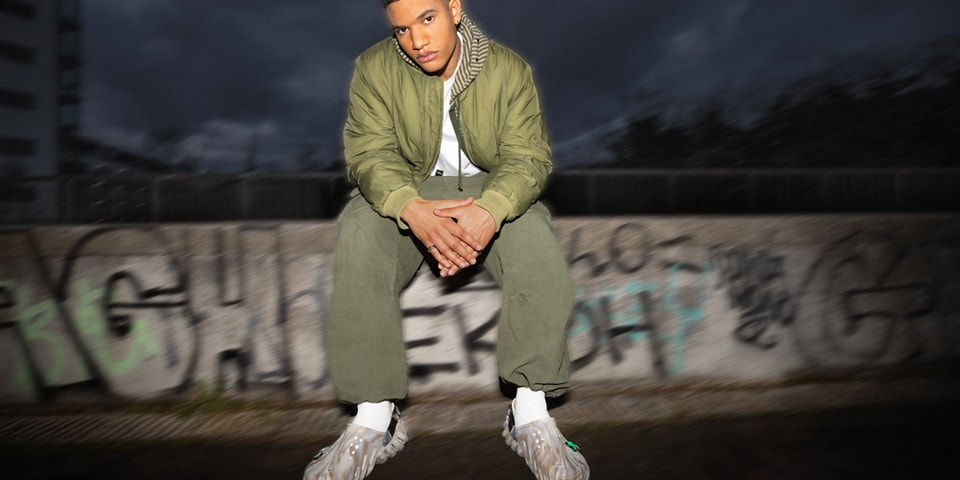This is a nighttime outdoor photograph of a young, light-skinned African-American male, likely in his late teens to mid-20s. He is sitting on a concrete wall or ledge that has graffiti, featuring letters like "A-G-H" prominently between his legs and "EK" and "OH" also visible. The man is wearing a medium olive-green jacket, a white shirt, matching green khaki pants, and marbleized Crocs with white socks. He has short dark hair and dark eyebrows, with his head slightly tilted to the left, looking straight ahead into the camera. The background is dark with clouds and possibly a building silhouette, but it is blurred, making the man the clear focal point. His hands, showing a black ring on his right pinky, are resting on his thighs. The overall setting is rather empty except for the detailed and vivid depiction of the young man illuminated by a strong light source, suggesting he might be photoshopped into the scene.